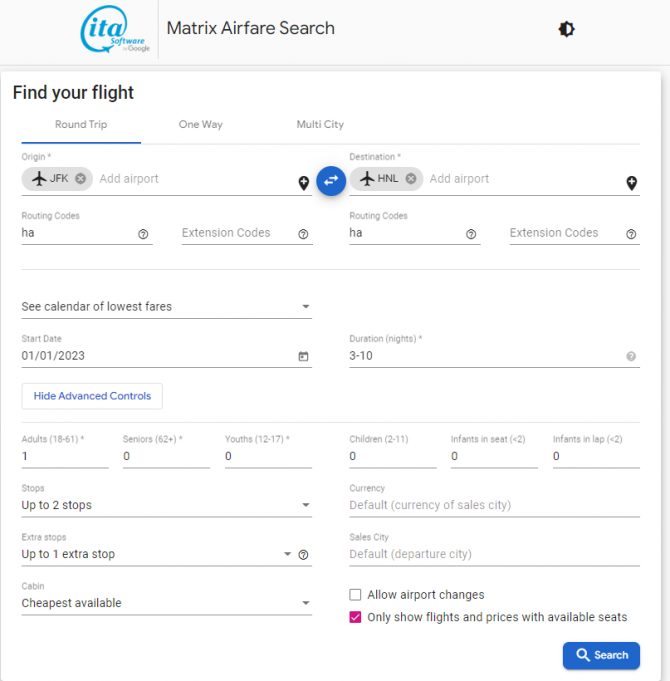This vertical image, captured from a web page on a computer or an iPhone, features an airfare search interface with a gray and white background. At the top, the title "EDA software from Google" appears in blue, followed by the black text "Matrix Air Force search" on the left, and a settings icon on the upper right. These sections are separated by a thin line.

Below the header, bold black text reads "Find your flight." The search options include "Roundtrip," "One-way," and "Multi-city," with "Roundtrip" being highlighted. The origin is set to "JFK," and the destination to "HLN." There are fields for routing codes and HA extension codes for both the origin and destination.

Further down, a calendar interface displays "Lowest fares," with a start date of "01-01-2023" and a duration of "3 to 10 nights." A button labeled "Hide advanced controls" is available to customize the view. The calendar is prominently visible, showing the lowest fares for various dates.

Passenger details are listed next, with categories for adults, seniors, youths, children, and infants in both seats and laps. Only one adult is selected, with all other categories set to zero. 

Flight preferences indicate options for up to two stops and up to one extra stop. The cabin selection is set to the "Cheapest available," with currency and sales city both set to their default values. An unchecked box labeled "Allow airport changes" is present, along with a checked box that says "Only show flights and prices with available seats." Finally, a blue button labeled "Search" is located at the bottom of the interface.